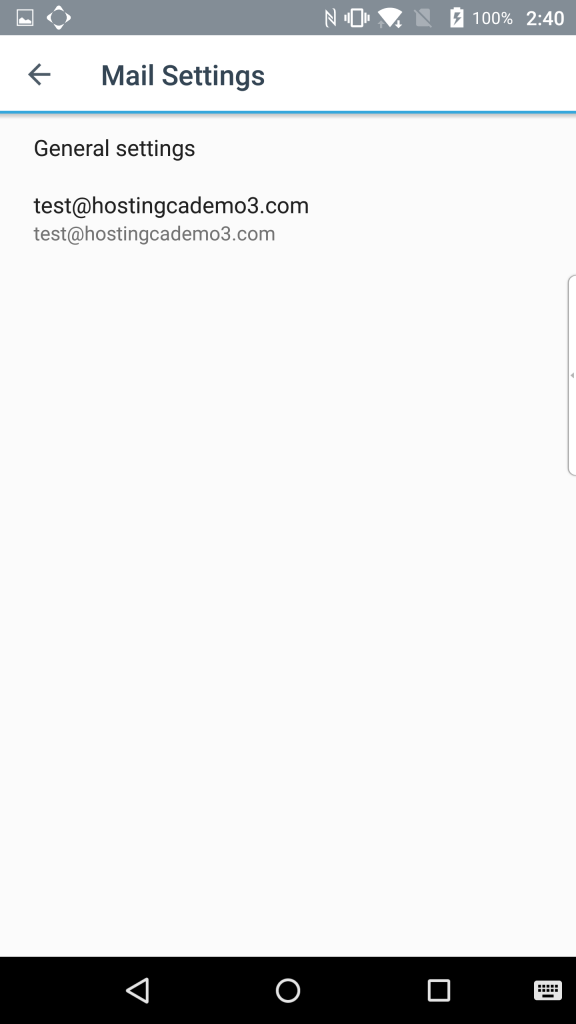The image depicts a phone settings menu page. At the top of the page is a long gray rectangle. Inside this rectangle, there is a box featuring a landscape at the bottom. Adjacent to this is a white square that appears rotated counterclockwise. In the upper right-hand corner of the screen, several icons are visible: the phone's vibrate symbol, the internet connection symbol, and the battery indicator showing 100% power. The current time is displayed as 2:40.

In the middle of the page, bold gray lettering reads "Mail Settings," accompanied by a left-pointing arrow. Below the "Mail Settings" heading is a thin blue line, followed by text that reads "General Settings" and "test@hostingcadmo3.com," repeated twice.

At the bottom of the page, a long black rectangle houses several navigation symbols: a left-pointing arrow, a circle, a square, and a keyboard icon.